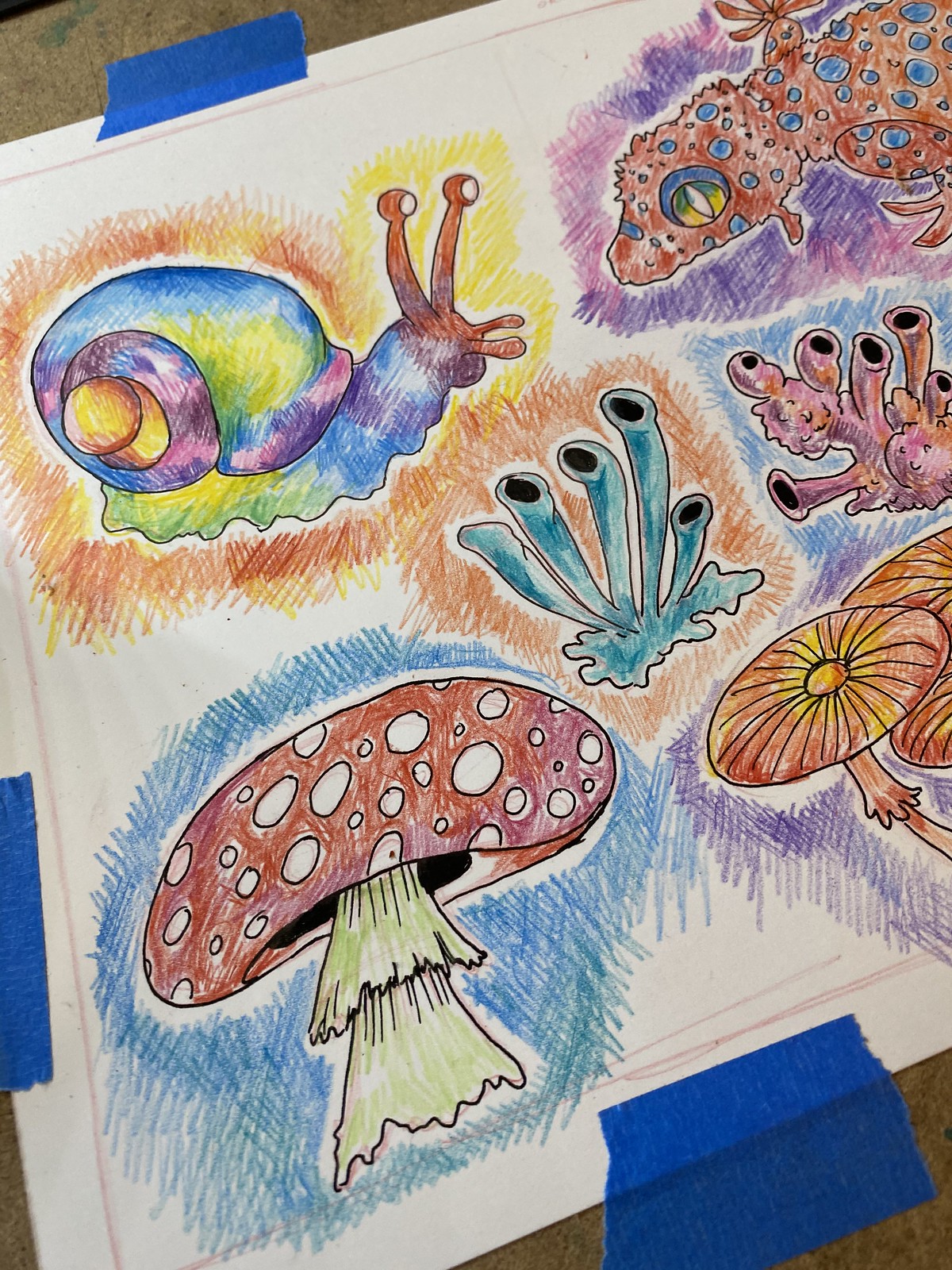The image is a vibrant, colored pencil illustration taped to a brown, clipboard-like surface using short, ripped pieces of blue painter's tape on all sides. The right side of the image is cropped out. At the top left, a snail with protruding eye stems features a multicolored spiral shell in shades of blue, green, purple, pink, and yellow, with a yellow and orange gradient shading around it. Below the snail are two tube-shaped fungi or coral-like structures—one predominantly blue with orange shading, the other light purple and orange with a blue outline. In the bottom left corner, a large red mushroom with white spots and a green stem is shaded with blue crosshatch to enhance its appearance. To the right of the large mushroom, more mushrooms with flat, red, and yellow tops are shaded in purple. In the top right corner is a reddish-brown gecko with blue spots, green-yellow eyes, and a purple shading. Additional mushrooms in the bottom right have taller, skinnier stems and flat circular tops, colored red and brown with purple shading. The overall composition emphasizes contrasting colors and detailed shading to make each element pop against the page.